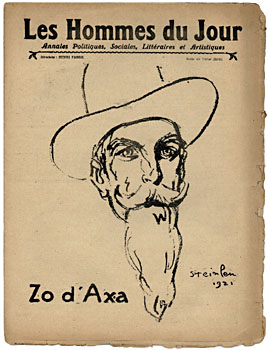The image depicts a tall rectangular, old-fashioned sign on a frayed, light brown parchment with visibly uneven and ripped edges, especially at the bottom and right sides, where the distress is more pronounced. The corners of the parchment are slightly curved. Dominating the center is a detailed, black ink sketch of an elderly man’s head. He is distinguished by his thick mustache, a very long narrow beard, and a tall cowboy hat. The man’s gaze is directed forward but slightly to the right.

At the top of the image, in formal, medium-sized black font, are the French words "LES HOMMES DU JOUR," followed by some smaller, indistinct words in black and a horizontal black line underneath them. Below this, to the left of the man’s substantial beard, is the text in bold black letters "ZOD’AXA." Adjacent to the right of the beard, in smaller handwriting, appears an artist’s signature, possibly reading "Steinman" or "Stein Lim," followed by the date "1921." The overall tone of the parchment suggests an aged, discolored look, contributing to its antique appearance, akin to an old advertisement or wanted sign.